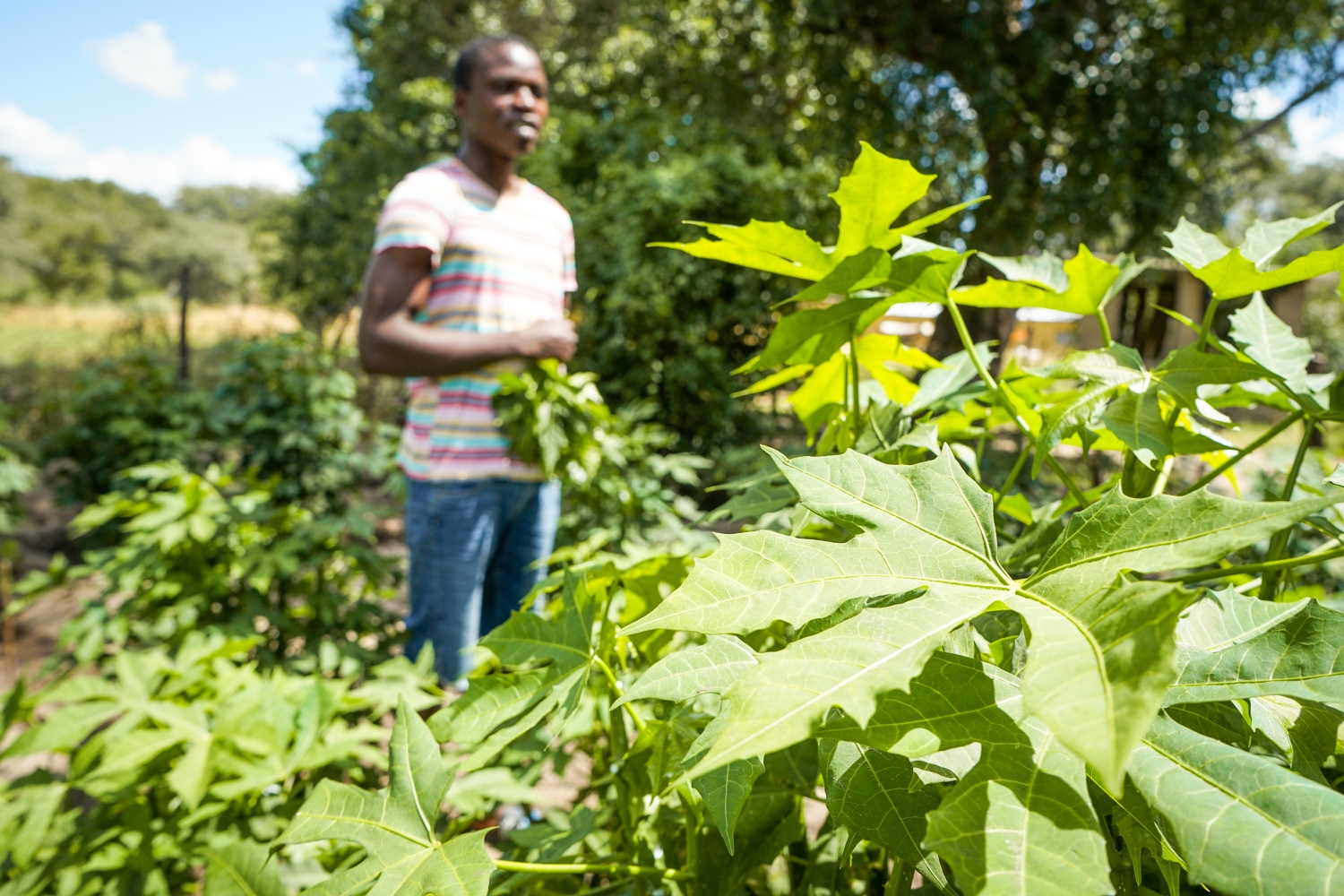In the image, there is a dark-skinned individual, likely African or African-American, with short black hair. They are standing in a field that resembles a farm, surrounded by green plants with jagged, spiky-edged leaves, possibly cassava or marijuana, as there are varying opinions about the plant type. The person is wearing a vibrant, short-sleeved, striped t-shirt with hues of blue, pink, yellow, green, and white, pairing it with blue jeans. They have one hand placed in front of their stomach and appear to be gardening or handling the plants around them. The background of the image features blue skies dotted with white clouds, numerous trees, and a blurry structure with a brown dirt ground.